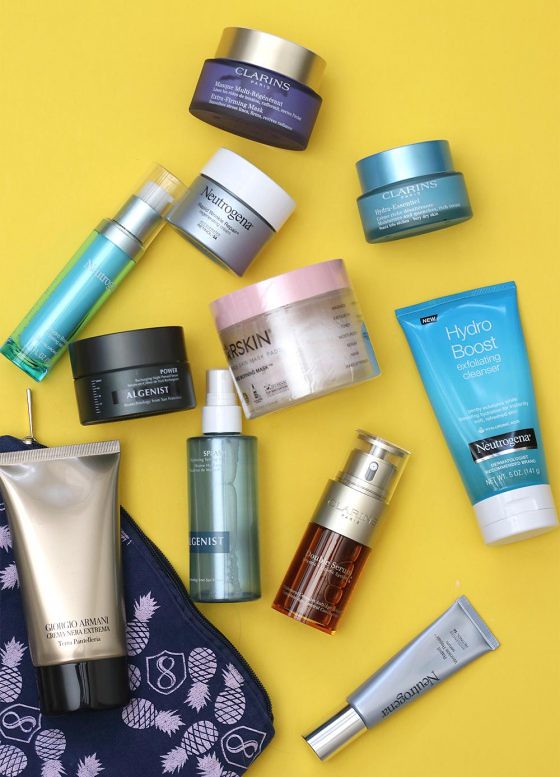The photograph showcases an array of health and beauty aid products meticulously arranged against a vibrant yellow backdrop, possibly a table. In the bottom left corner, there's a navy blue zip-up makeup bag adorned with a pattern of small white pineapples and a shield symbol bearing the number 8. Resting atop the bag is a product housed in a sleek, metallic squeeze tube with a black cap. 

Sprawled across the yellow surface are various other beauty products, including a slender Neutrogena silver tube with a matching silver screw cap. Another standout item is the Neutrogena Hydro Boost product, which features a striking turquoise body paired with a white flip cap. The Neutrogena logo is designed in black with white lettering.

Above these, there's a small jar by Clarins, entirely in a soft blue hue, with white font accents. Positioned adjacent is another jar from Clarins, rendered in a slightly darker blue shade. Additionally, the display includes three smaller pots varying in size and color. One is from Algenist, another from Neutrogena, and the third appears to be labeled "Clear Skin." These pots come in pink, silver, and black.